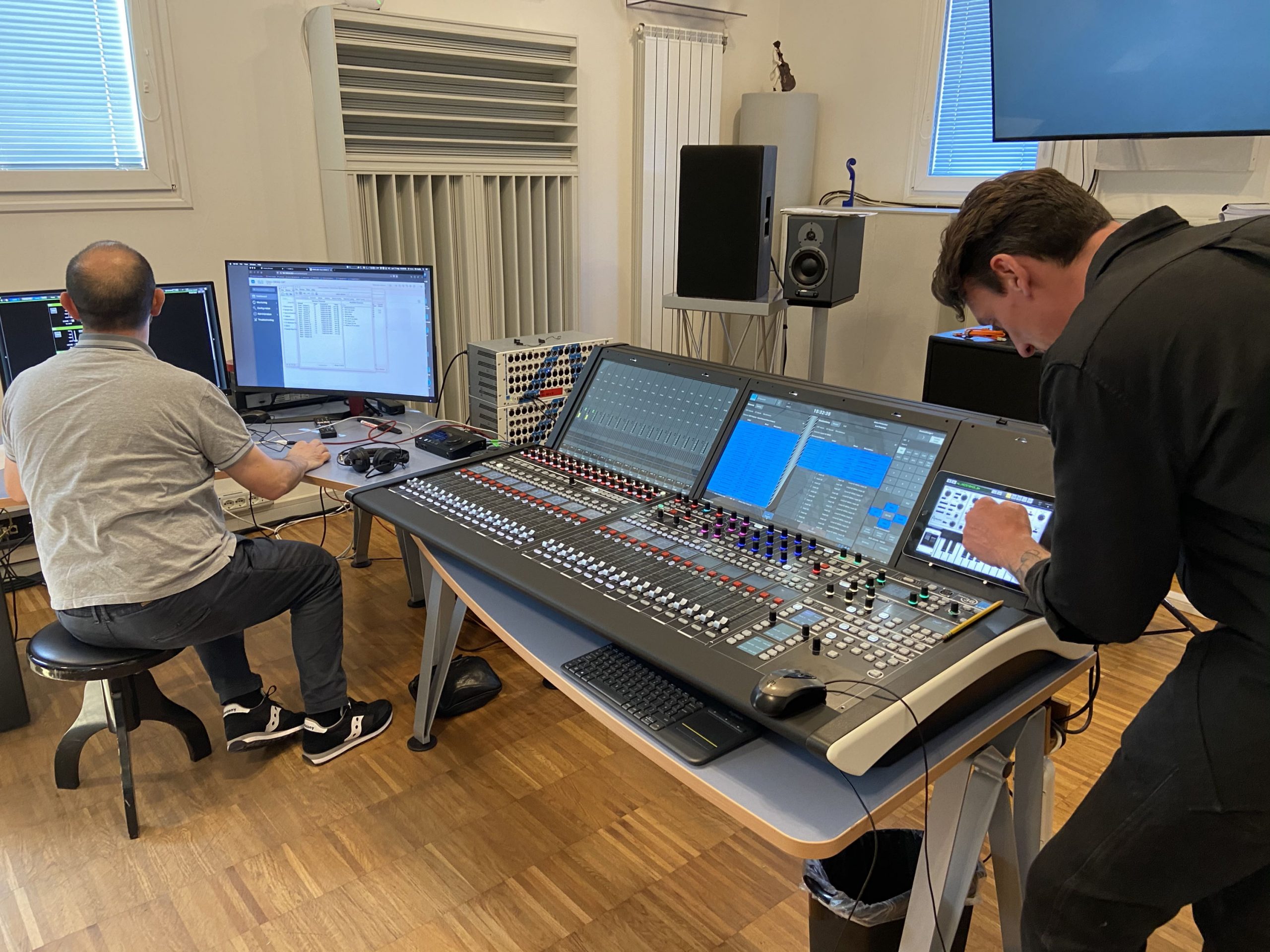In this detailed photo of a music studio, two men are present. The man on the left, dressed in a grey shirt, dark grey pants, and black shoes, is seated on a three-legged stool with his back facing us. He is focused on adjusting or editing content on two computer monitors positioned in front of him on a gray table. Adjacent to him, towards the middle of the image, is a large electronic contraption featuring numerous knobs, dials, and push buttons. The second man, dressed in all black, is bent over this device, seemingly at work. The room itself has off-white walls, and its acoustics are enhanced with baffles on the wall. Large speakers are strategically placed throughout—both on stands and platforms—while a ceiling-mounted monitor and an overhead projector are also visible. The floor is a light-colored wood, potentially tiled. The blinds in the room are closed, and there’s a garbage can under the table, along with visible cords hanging from the soundboard.